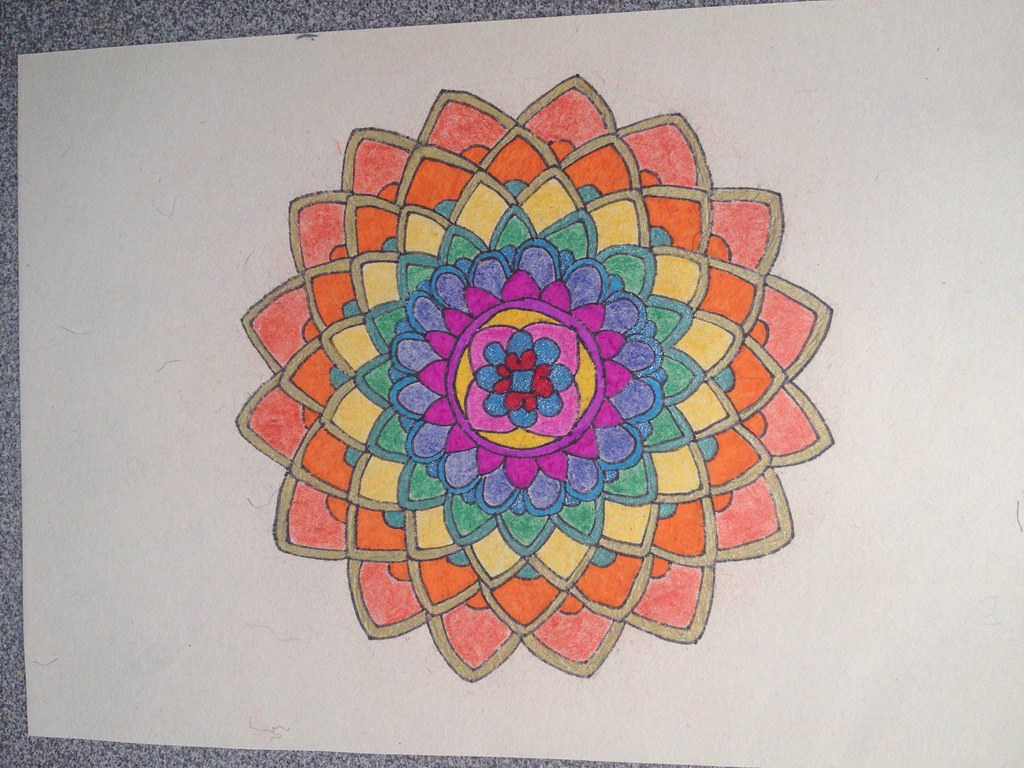The image presents a highly detailed, hand-drawn mandala on a white sheet of paper, which is positioned horizontally on a grayish carpet. The mandala itself is a complex arrangement that maintains its symmetry regardless of its orientation, reminiscent of a kaleidoscope. 

At its core, a blue flower with a red center and a purple base anchors the design. Around this central motif, eight layers of meticulously detailed petal shapes radiate outward, creating a 3D effect. The first layer features a pattern of red petals, followed by blue, purple, yellow, and another purple circle, with progressively larger sets of petals in varying shades including green, light purple, and light blue. The outer layers include light orange and deep orange star-like shapes, pastel yellow, bright pink, and finally, fringe details in green and lighter green.

The combination of geometric precision and vibrant colors in this mandala offers a visually captivating experience, akin to viewing a static image inside a kaleidoscope.